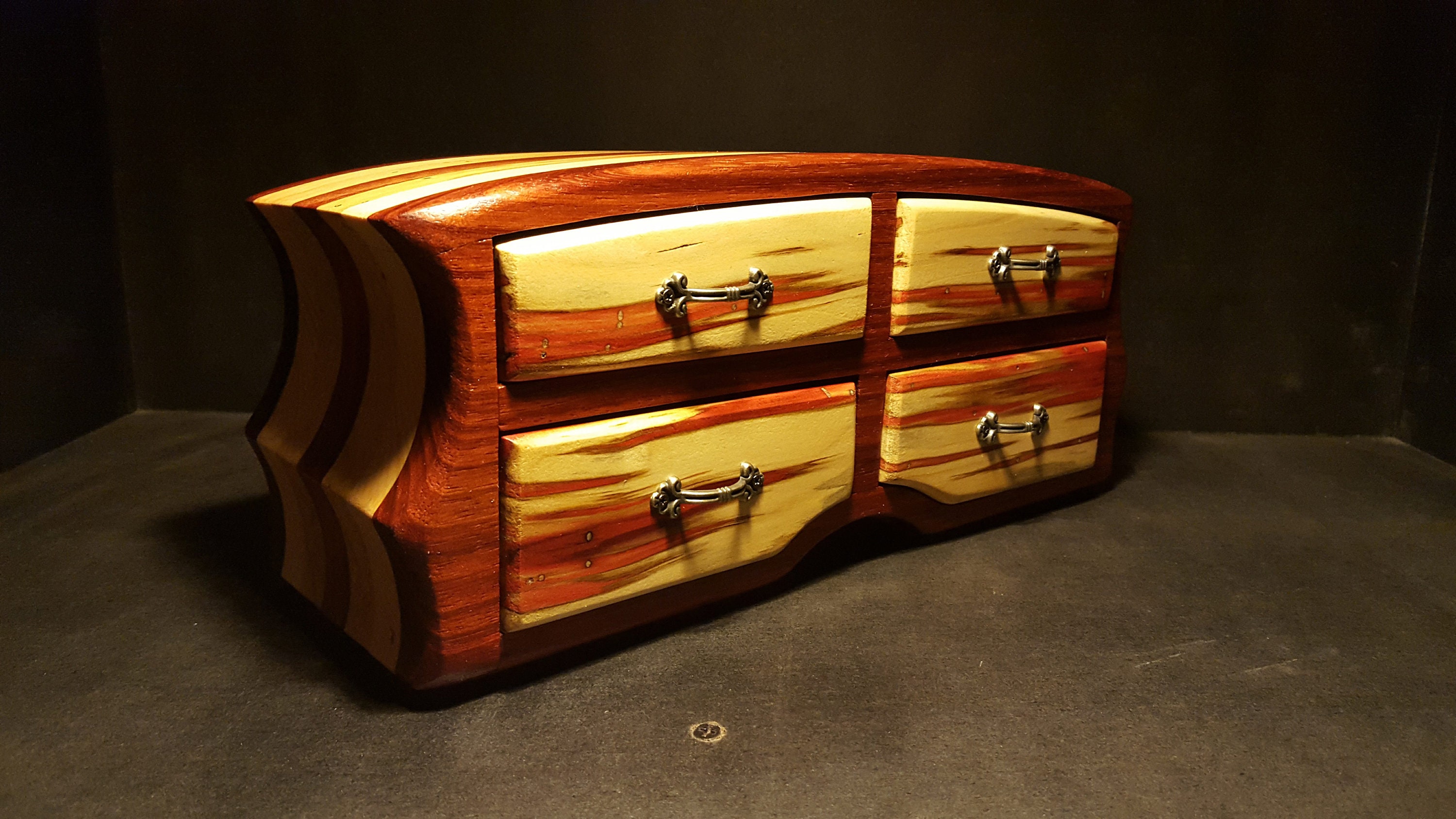The image depicts a unique piece of furniture resembling a chest of drawers or jewelry box, characterized by its distinctive curvilinear design and dual-tone wood finish. The top surface of the chest is arched, transitioning into a convex curve before narrowing and then flaring out again towards the base. This curvy silhouette gives the impression of a sculpted, undulating form reminiscent of a bitten cake. The chest features four rectangular drawers, each adorned with silver pull handles. The wood is an eye-catching combination of dark brown and light yellow tones, with the darker wood framing the perimeter of the drawers and extending seamlessly across the top. The setting is austere, placed against a backdrop of dark gray cement walls and floor, which includes a small floor drain. The contrast of the dark background and the furniture’s dark base enhances the chest's polished and artistic appearance.